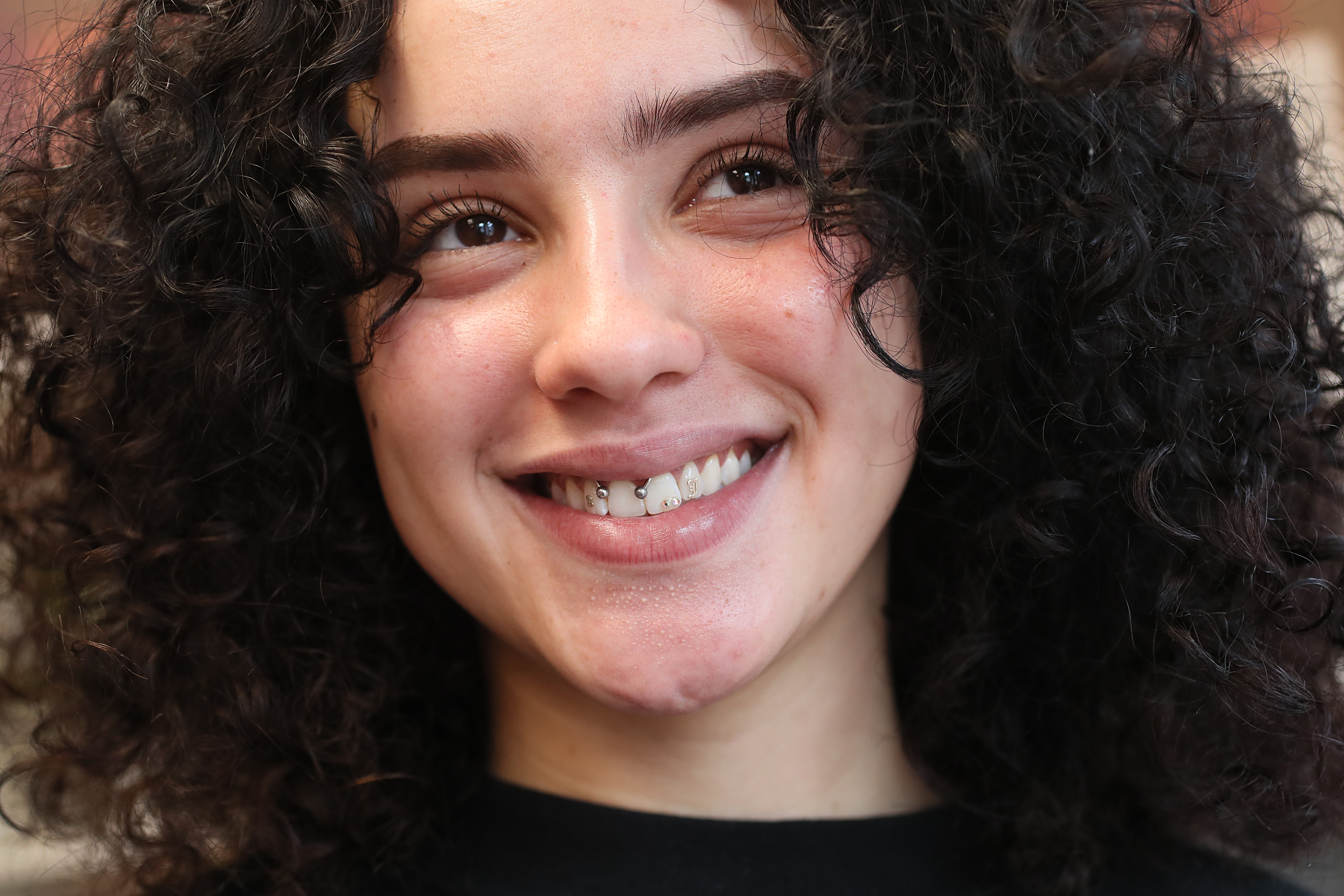This image is a detailed close-up portrait of a young woman, most likely in her teenage years. She has dark, curly, frizzy black hair and prominent, thick, well-groomed eyebrows. Her eyes, which appear to be brown, are looking upwards and to her left. She has long eyelashes that accentuate her bright and pleasant expression. The woman's face dominates the frame, which cuts off part of her forehead and her head just below the neck, revealing she is wearing a black top. 

Her smile is wide and warm, revealing unique dental features: between her two front teeth and also between the second and third tooth on her left, there are small silver balls. Additionally, her right front tooth has two metal bars at the gum line, adding a decorative or possibly functional element to her smile. Dimples frame her smile, including a notable dimple on her chin, further enhancing her cheerful appearance. The background is not visible due to the close-up nature of the photograph, focusing all attention on her expressive face and distinctive features.